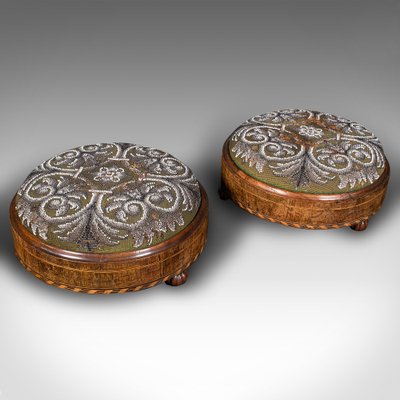This photograph features two nearly identical, round objects positioned side by side on a white surface, set against a background that shades from a light pewter at the top to white at the bottom. These objects have polished wooden sides with a rich mix of dark and light brown tones, suggesting a handcrafted element. They appear to have three wooden peg legs each, elevating them slightly above the surface. The tops of these objects are upholstered with an olive-green fabric, adorned with a white, chalk-like sketching that forms a diamond pattern in the center and four circular motifs positioned at the 12, 3, 6, and 9 o'clock positions. While their exact purpose is unclear, they resemble either jewelry boxes or ottomans, and are designed to hold delicate items or serve as footrests.